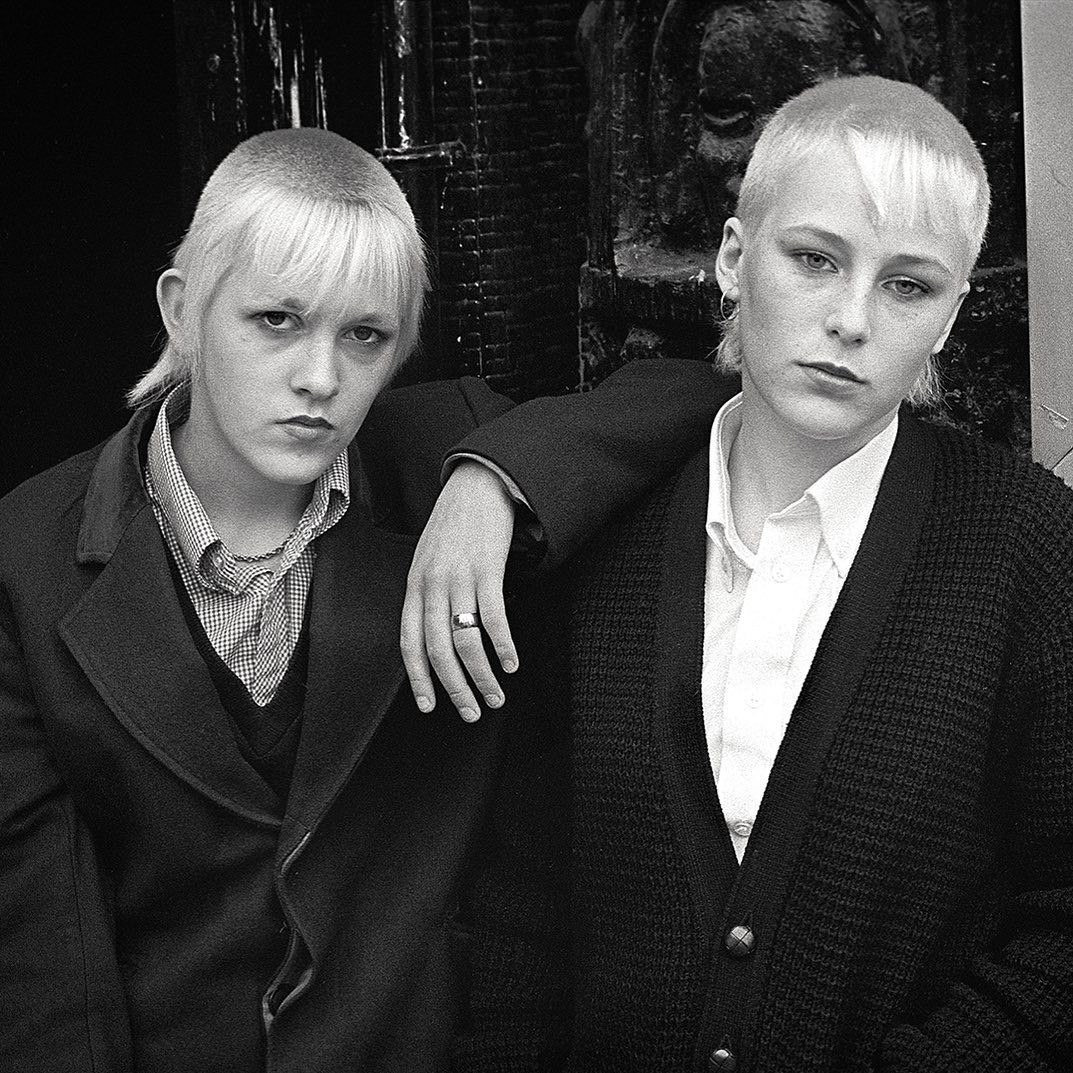This black-and-white photograph captures two individuals standing outdoors in front of a stone fountain with a face carved into it, set against a brick wall. Both individuals sport very short, fair hair cut into a mullet variation, with shaved sides, intact bangs, and some hair sticking out at the back. The person on the left is wearing a dark peacoat over a sweater vest and gingham shirt, while the person on the right is dressed in a heavy, knitted cardigan over a light-colored button-down shirt, accessorized with an earring in the right ear. They stand close together, with the left person's left arm resting on the right person's shoulder, revealing a thick, possibly gold wedding ring on the ring finger. Both individuals gaze at the camera, the left with a slightly more intense look than the right. Despite the photograph's monochrome palette, it captures the detailed textures of their clothing and the serene, perhaps contemplative, expressions on their faces, along with a backdrop suggesting a tranquil outdoor setting.